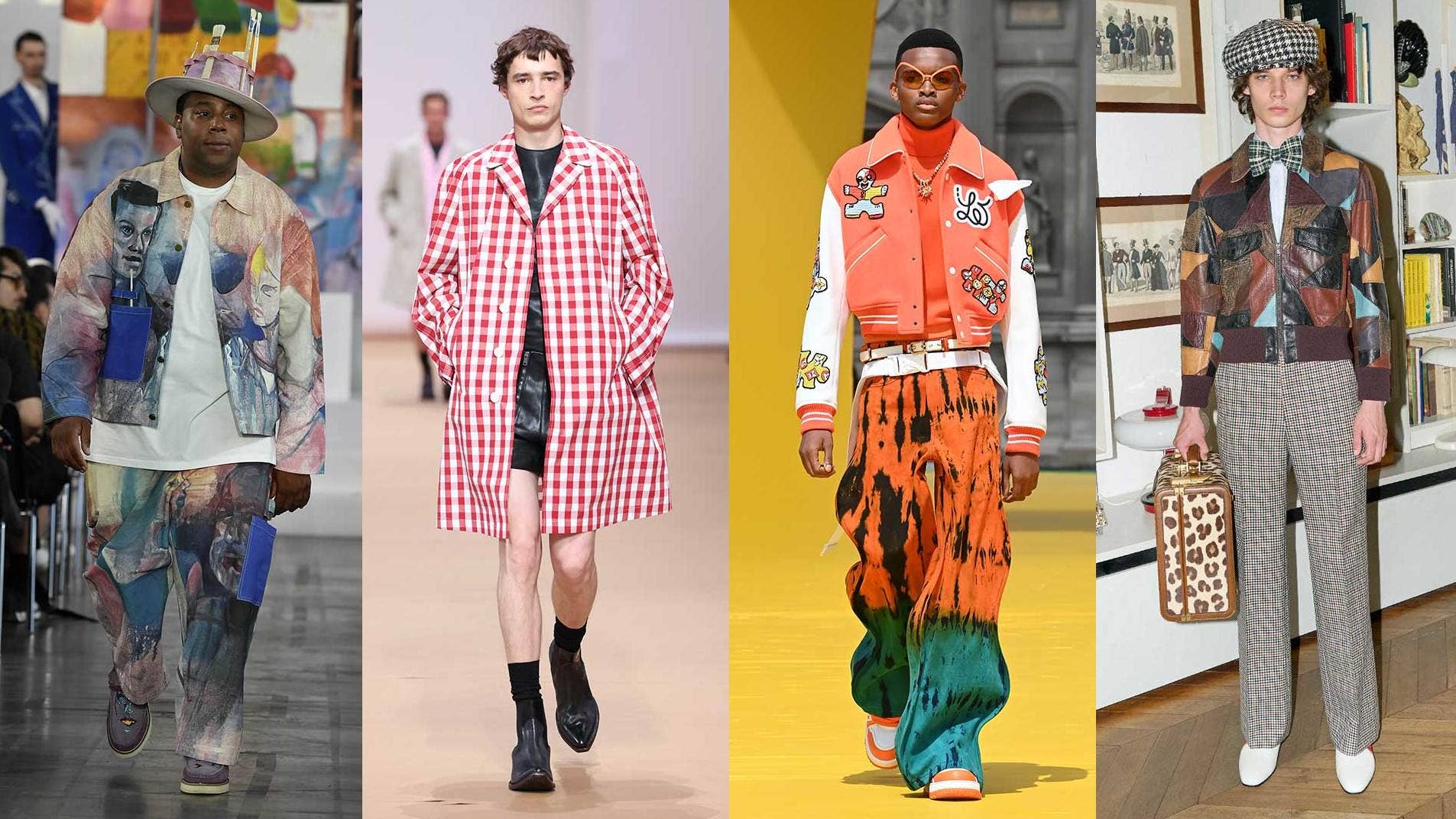This composite image showcases four distinct fashion looks modeled by male models, featuring diverse styles and vibrant colors. 

On the far left, a black model, possibly Kenan Thompson, strides down the runway wearing a white t-shirt under a tan jacket adorned with abstract faces reminiscent of graffiti. He pairs this with matching pants, a hat embellished with paintbrushes, and purple-gray loafers. 

Next, a white model dons a red gingham coat over a shiny black outfit that includes very short shorts. His ensemble is completed with black leather shoes and dress socks. Another model trails behind him on the runway, partially visible. 

The third image presents a black model sporting an orange varsity jacket with white sleeves, orange-tinted sunglasses, and striking orange and blue tie-dyed pants. His footwear consists of orange sneakers, likely Nikes, adding a cohesive touch to his bold look. 

The final model, on the far right, is a white man posing in front of a decorative bookcase rather than walking the runway. He wears a checkered hat and bow tie, a leather jacket made from various colored patches—blue, black, orange, yellow, and brown—plaid pants, and white leather shoes. In his hand, he holds a cheetah-print suitcase, adding an element of wild flair to his eclectic ensemble.